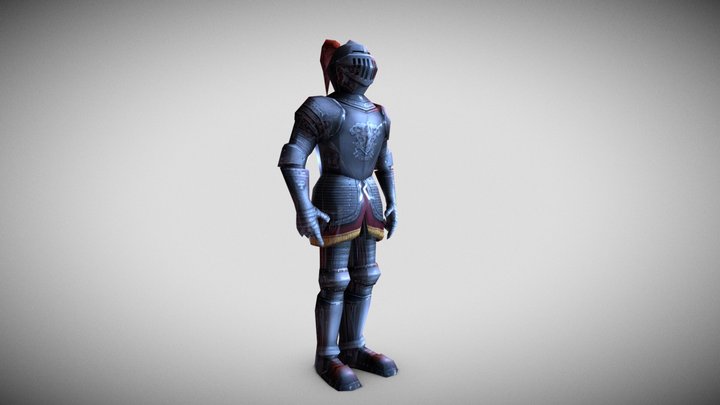The image is a 3D illustration of a medieval knight set against a gradient gray background that transitions from light gray at the center to dark gray and black at the corners, creating a shadow-like effect. The knight, positioned at the center and facing the bottom right, is depicted in a semi-pixelated, cartoonish style with a steel blue hue to its armor. The knight's attire includes a helmet and full arm and leg armor. Its chest plate is gray, and it wears red sabatons paired with gray greaves. A red skirt with gold edging adorns the lower section beneath the chest plate. Notably, the knight features a red ponytail extending from the back of the helmet. The shadows around the knight, particularly around the shoulders and legs, enhance the 3D contours of the figure, emphasizing the detailed rendering of the armor.